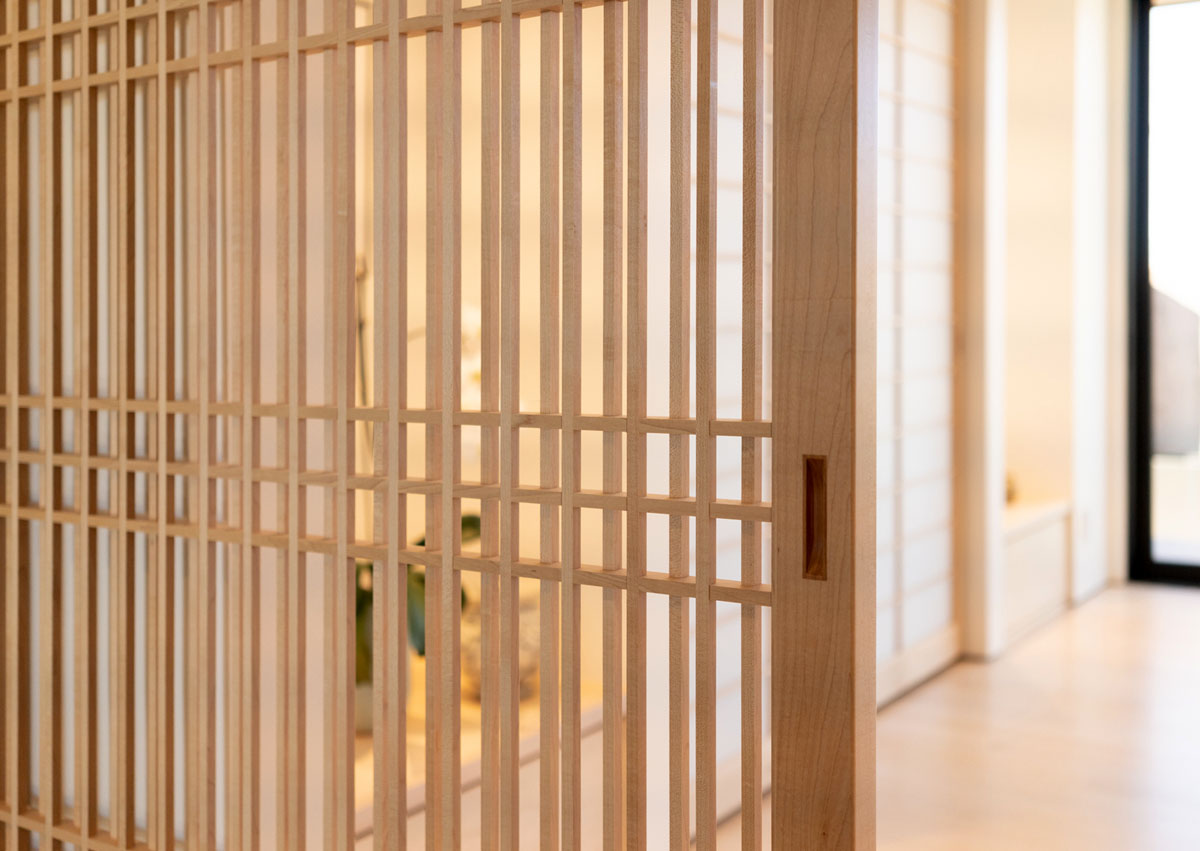The photograph captures an interior scene of a house, featuring a prominent sliding wooden door or gate adorned with a configuration of vertical and horizontal slats. This door, which has a light wood color, spans two-thirds of the photo from a vertical angle and resembles the design of closet sliding doors. Through the slats, one can see a blurry background, possibly showcasing a room lit by either natural or artificial light. To the right of the sliding door, there's a hallway and a partial view of a black-framed door or window, mostly visible from the top right corner, extending about 70-75% downwards. The surrounding walls appear to be white, contrasting with the tan or brownish wooden floor. In the background, details are indistinct, but there seems to be a hint of a person sitting on the floor, along with some items such as a large window or possibly a door with glass panels, a white object which could be a toilet, and a plant with a green flower in a white pot, adding a touch of greenery to the scene.